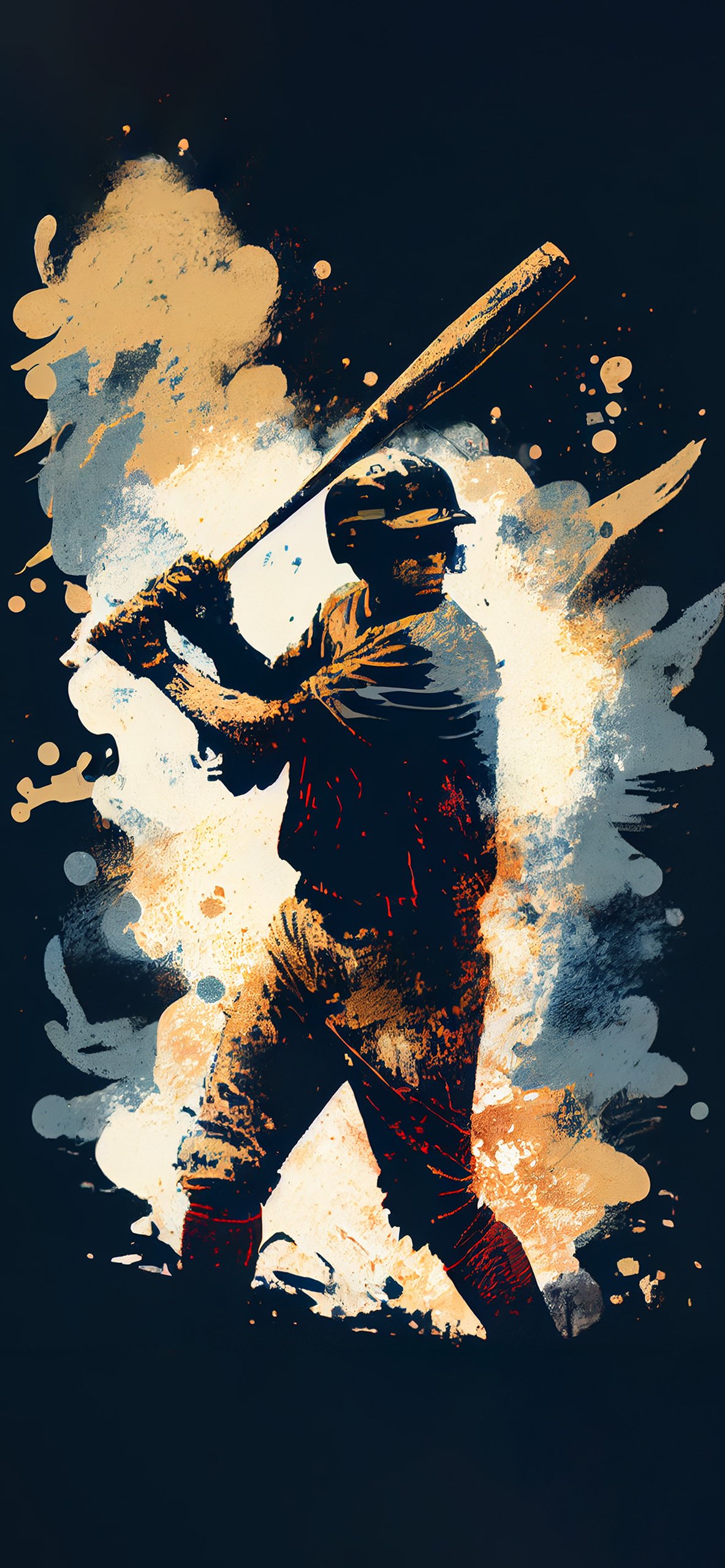The image showcases a vertically rectangular print with a stark black background. Splashes of white, gray, light brown, and tan paint create a splotchy, artistic backdrop. In the foreground stands a baseball player, centrally positioned, ready to swing a bat poised above his head. He is equipped with a helmet and a pair of gloves, and sports a multicolored uniform featuring hues of yellow, red, blue, and rust. The player is facing towards the right side of the image. The bat he holds is a combination of black and yellow, and his uniform pants are cinched at the waist, with the rust-colored socks extending past his knees. The detailed representation captures the dynamic energy of the player through an artistic style that could be either watercolor or digitized artwork.